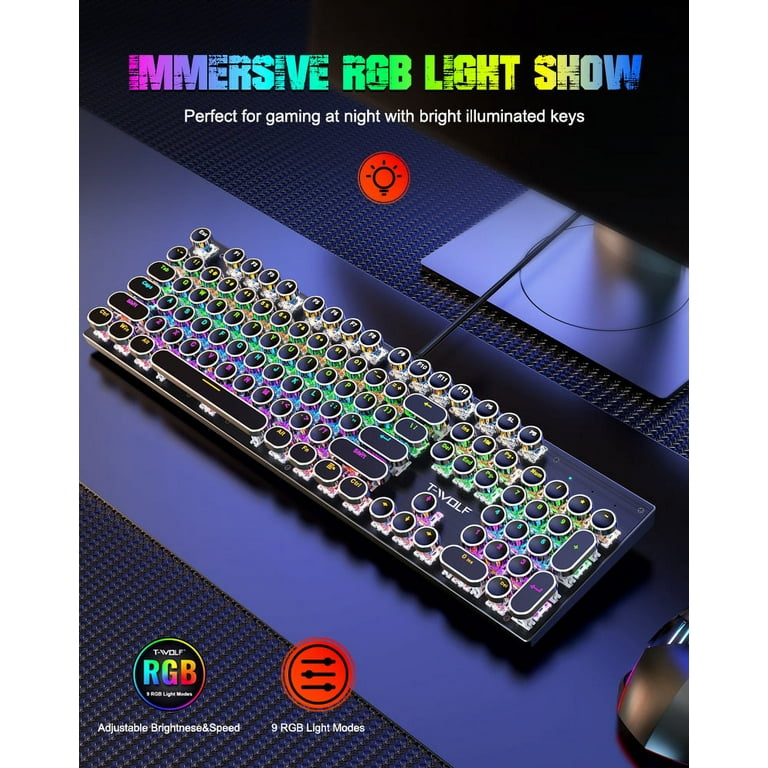This advertisement showcases a sleek, black gaming keyboard from T-Wolf, designed with round, bubble-like keys and RGB lighting. The keys are vividly illuminated in a spectrum of colors, including green, blue, purple, yellow, and white, creating an immersive RGB light show perfect for night gaming. The top of the ad features "Immersive RGB Light Show" in vibrant, changing neon letters, followed by "Perfect for Gaming at Night with Bright Illuminated Keys" in white text. Below this, a red circle with a white light bulb symbol emphasizes the lighting feature. At the keyboard's base, the T-Wolf logo is accompanied by the text "RGB Adjustable Brightness and Speed." To the right, another red circle highlights "9 RGB Light Modes" with black slider icons. The keyboard is set on a blue-silver desk with a mouse positioned to the right.